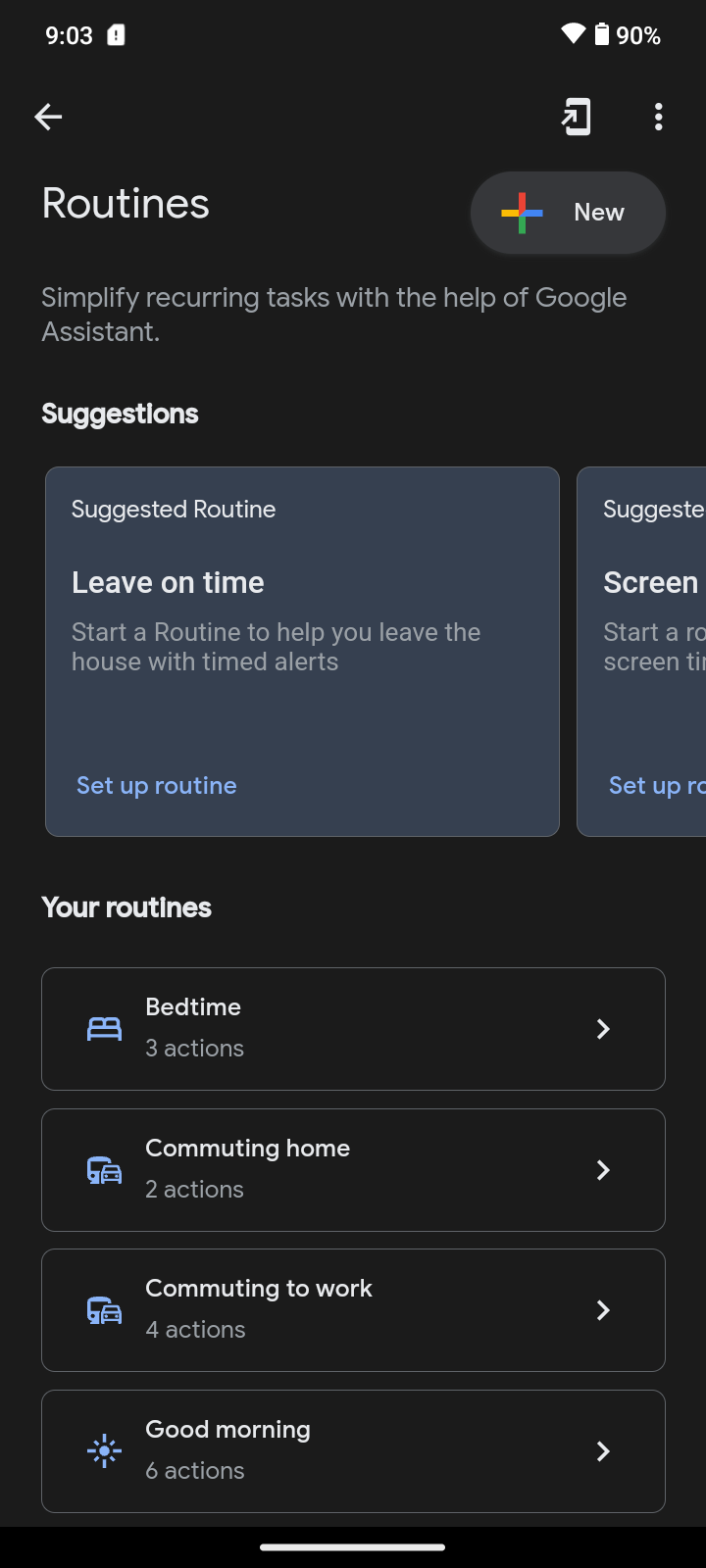Screenshot of a Google Assistant interface showing the "Routines" section at 90% completion. The interface prominently features a multi-colored Google symbol in the shape of a plus sign, with each of the four lines in red, blue, green, and yellow. The header reads, "New: Simplify recurring tasks with the help of Google Assistant."

Below the header, there are suggested routines including:

- **Leave on Time:** Start a routine to help you leave the house with timed alerts.

Additional options include setting up new routines and viewing existing ones, such as:

- **Bedtime:** 3 actions
- **Commuting Home:** 2 actions
- **Commuting to Work:** 4 actions
- **Good Morning:** 6 actions

Each section features a right-pointing arrow for further navigation. A light gray bar is visible at the bottom center of the screen, likely for additional options or information.